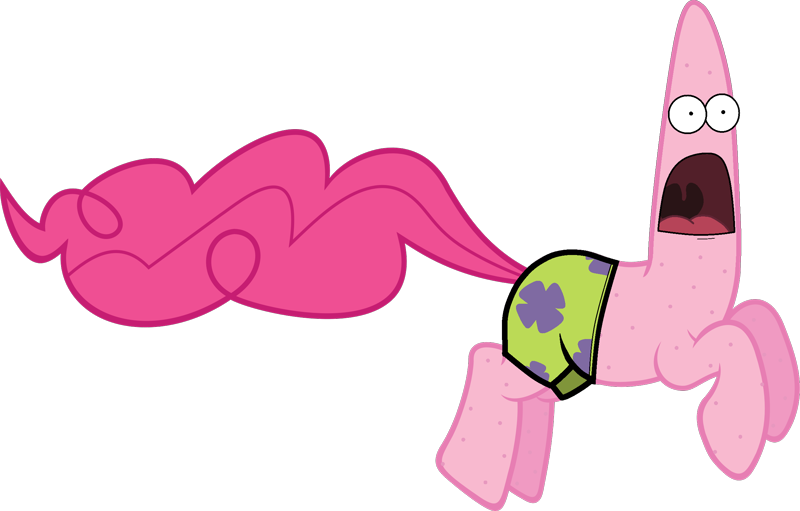This is a highly detailed and imaginative drawing of Patrick Star from Spongebob Squarepants reimagined as a unicorn in the style of My Little Pony. Patrick's head is distinctly cone-shaped, extending vertically before angling back down, with a half-oval, enormous open mouth revealing a pink tongue with a darker shade lining inside and a black shadow suggesting the throat. His expressive, very wide eyes are placed close together and feature large white sclera with small black pupils. His entire body is a vibrant pink with scattered dots, transitioning to a horizontally oriented equine form complete with four horse-like legs poised as if in mid-gallop. Patrick is wearing his signature lime green shorts adorned with a black outline and purple cloverleaf patterns. A long, flowing, and puffy tail in a hot pink hue, highlighted with darker pink swirls, trails behind him, adding a whimsical, animated flair similar to that of a My Little Pony character.